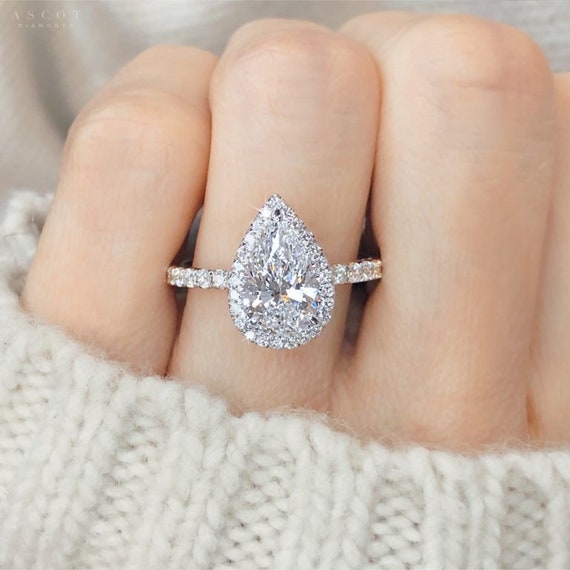This image features a close-up of a left hand with a pale complexion and a soft white sweater sleeve coming down to the knuckles. The hand is slightly bent to emphasize the focus on an engagement ring. The ring, set on the fourth finger, showcases a prominent upside-down teardrop-shaped clear stone, which could be Cubic Zirconia or Moissanite, surrounded by smaller stones. The band itself also features stones, although it is unclear if the entire band is adorned or just the upper portion. The intricate design sparkles with a silver sheen, accentuating the pointed and rounded facets of the main stone, reminiscent of a Ouija board pointer. The background is light, enhancing the hand and ring’s visibility, and in the upper left corner, a watermark reads "Ascot Diamonds," reinforcing the association with fine jewelry.